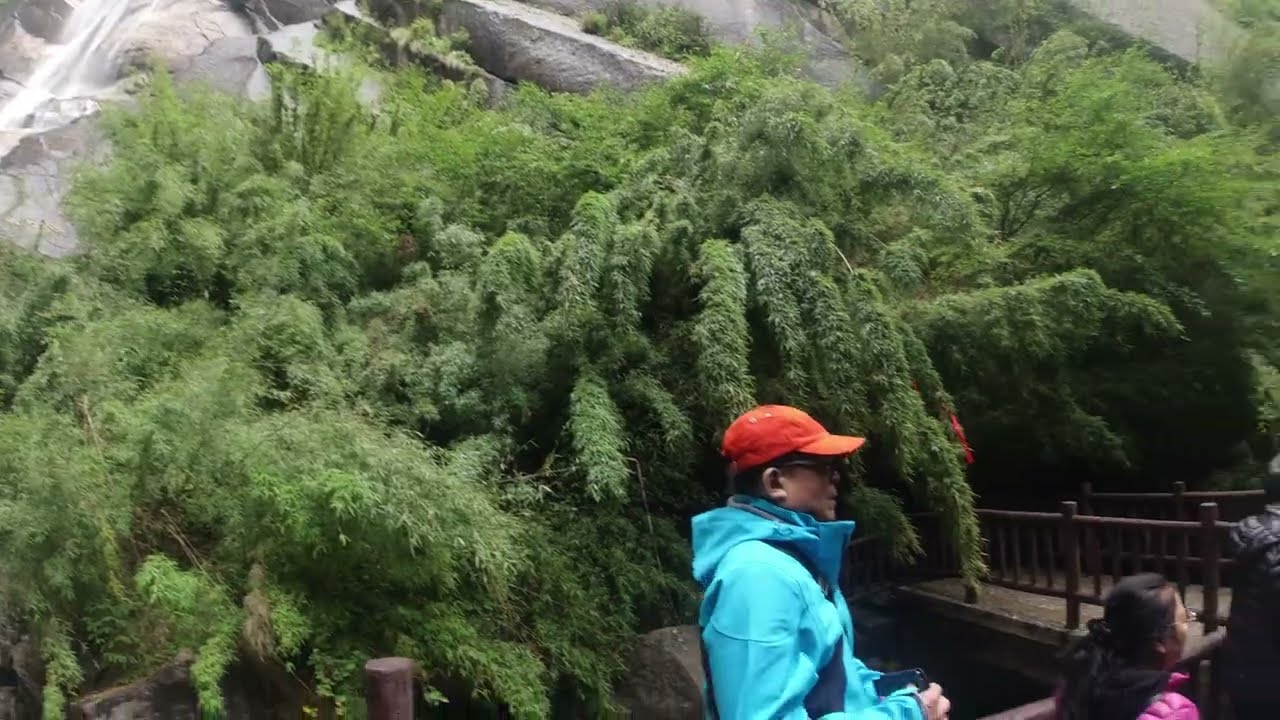In this vibrant photograph, an Asian man stands out in the middle, wearing a striking orange baseball cap, black sunglasses, and a vivid turquoise blue coat with dark gray accents. He holds a dark gray mobile phone in his right hand, suggesting he might be capturing the moment. To his immediate right is a young woman with long dark hair, styled and pulled back, wearing eyeglasses and a pink puff coat. Both are looking to their right. In front of the woman, and partly obscured, is another person clad in a black puff coat.

The scene is set on a bridge or walking path, constructed from dark wood and cement, blending seamlessly with the lush surroundings. The background is dominated by dense greenery with thick, bushy leaves and long, floppy tree branches. Wispy, heavy vegetation and possibly even bamboo create a serene, immersive nature trail ambiance. Towards the top of the image, a glimpse of rocky outcliffs adds to the rugged natural beauty. It's daytime, and the overall feel is one of tranquility and connection with nature, as the four individuals navigate the scenic pathway.